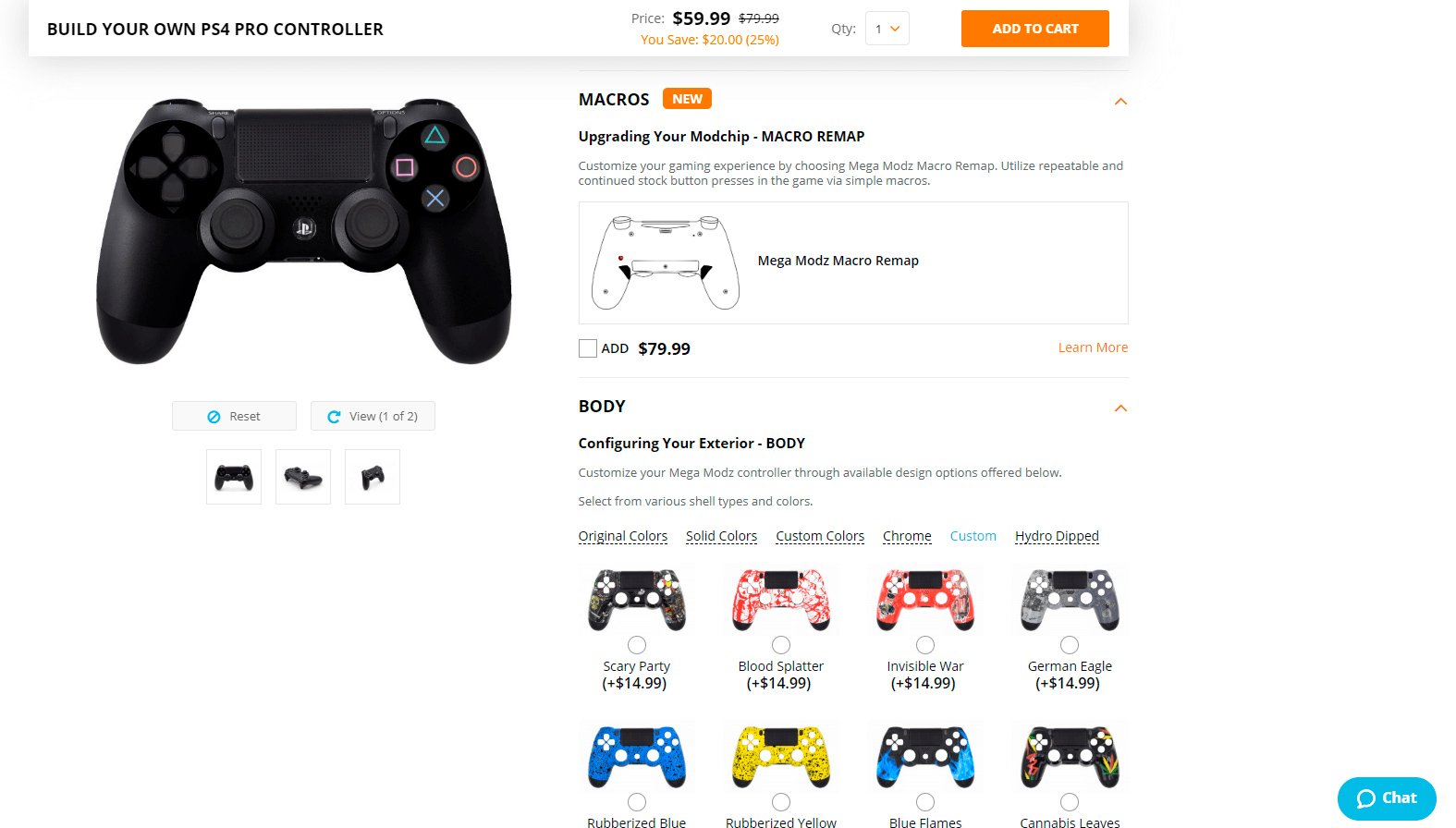This is a detailed screenshot from a website offering a customizable PS4 Pro controller. The upper left corner features a white background with black font text that reads "Build Your Own PS4 Pro Controller." To the right, the price is listed as "$59.99," with a note below indicating that you save "$20.25." The quantity is set to "1," and there is an "Add to Cart" button in white font on an orange rectangle.

On the left side, there is a photo of a black PS4 controller, which appears identical to a standard PS4 controller. Below the image, there are two buttons labeled "Reset" and "360 View," allowing for customization and interactive viewing of the controller. Further down, there are three additional clickable thumbnail images of the PS4 controller for more detailed views. Below these images is a blank white rectangular area.

On the right side of the screen, additional information is provided. At the top, the word "Macros" is displayed in black font, accompanied by an orange rectangle with the word "New" in white font. Below this, it reads "Upgrading Your Mod Chip," suggesting more details about controller enhancement options.